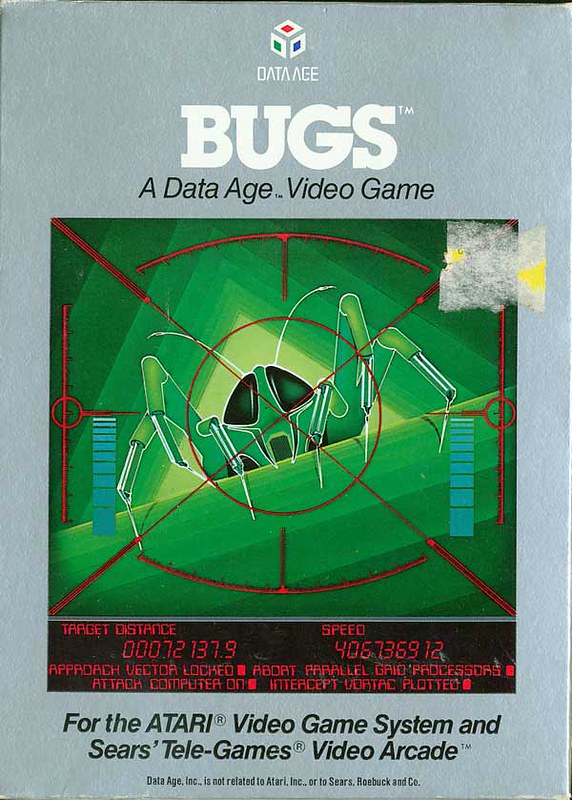The image features a vintage Atari video game box titled "Bugs," produced by Data Age. The box art prominently displays an in-game screenshot, showcasing red crosshairs zeroing in on a green spider. The spider sits against a textured green and beige background, accentuating the targeting aesthetic. At the bottom of the screen, targeting information suggests a scope view. The packaging highlights compatibility with both the Atari video game system and Sears Telegames Video Arcade. The well-worn box retains remnants of a price sticker near the top right corner. Overall, the box is shaded in a grey-blue hue, enhancing its retro appearance.